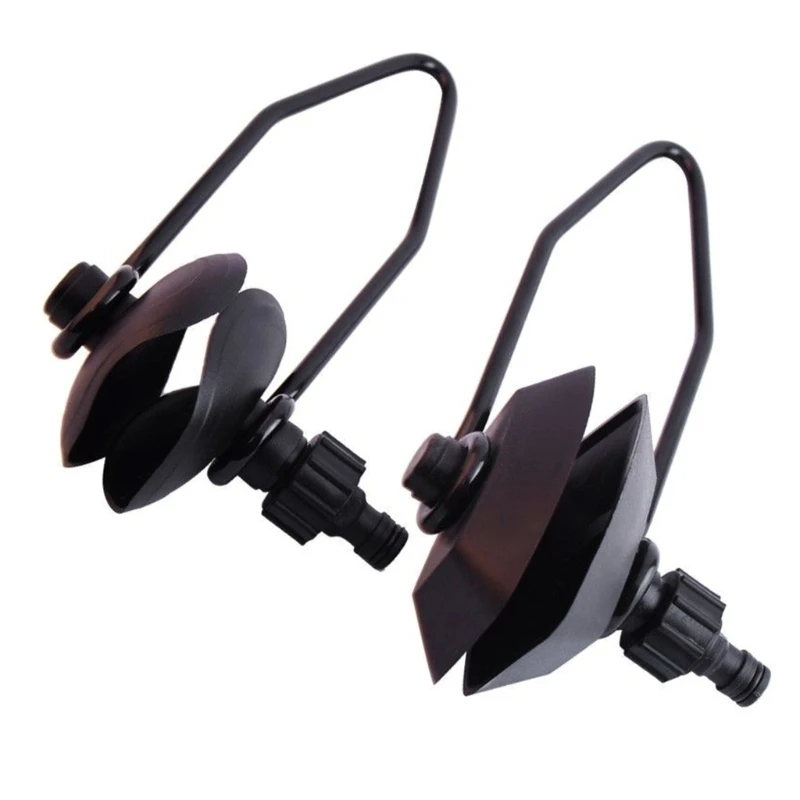This photograph showcases a pair of black clamping devices, arranged diagonally against a white or transparent background. The upper clamp features a rounded design reminiscent of headphones, with two paddle-like parts that can be tightened by a spinning black wheel. The lower clamp is more angular and square-shaped, with a flat section in the middle. Both clamps are constructed from dark to black materials and are equipped with a black bar and a threaded wheel mechanism for adjusting grip. The clamps exhibit intricate detailing, including a glossy finish and metal arms connected by black wires that provide structural support and functionality.